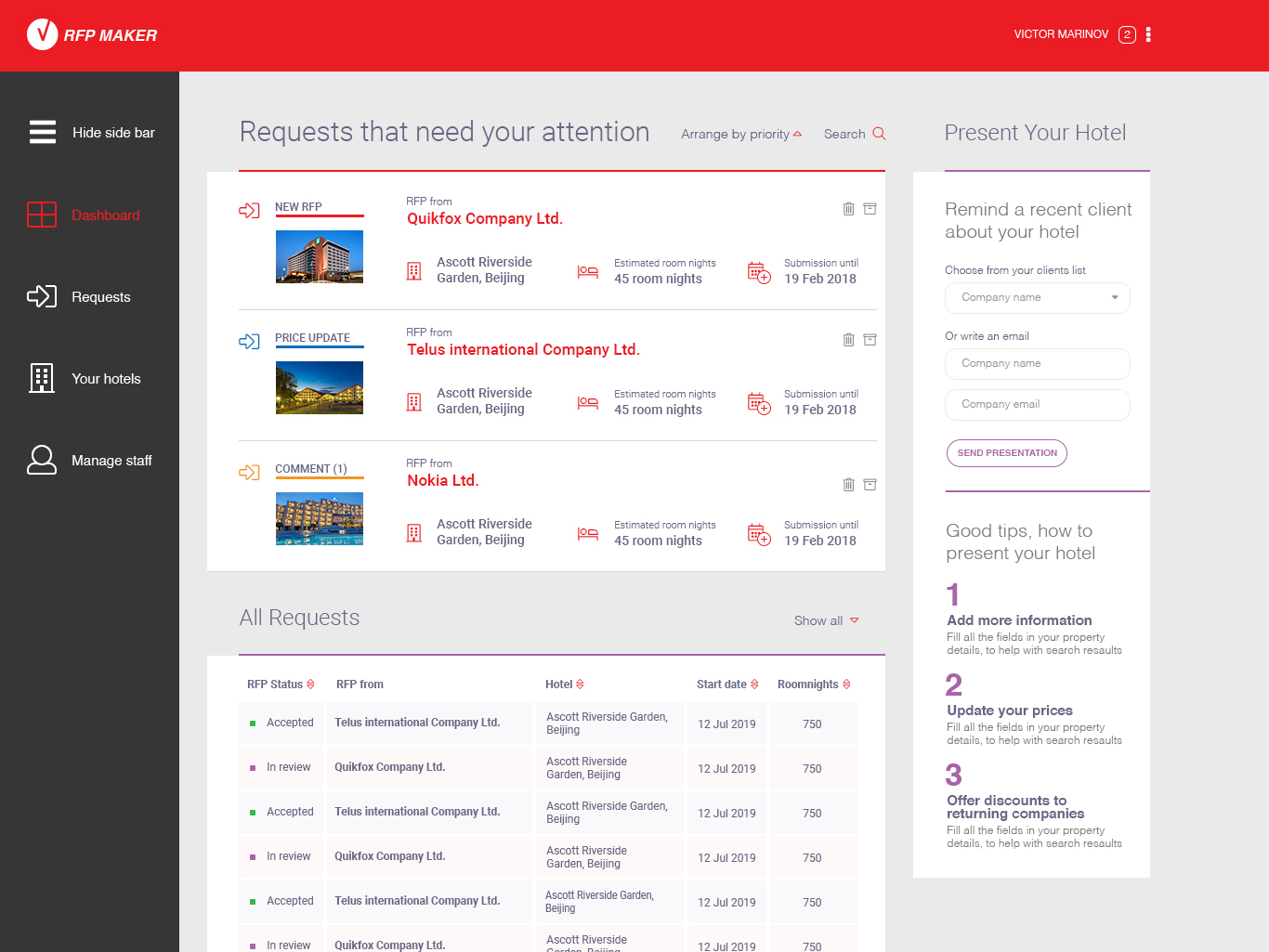This screenshot captures a user interface from a hotel management application named RepMaker. At the top-center of the image, a red box prominently displays the application's name, "RepMaker," with the user name "Victor Manitow" visible on the top-right corner. To the left, a dark gray sidebar contains a button labeled "Hide Sidebar," and directly below that, in red text, it reads "Dashboards."

In the main section of the screenshot, there is a header that states "Request to your Hotel's Managed Staff" followed by a sub-header "Requests that Need Your Attention." The first request listed is from QuickFox Company, LTD based in Beijing, which requires an estimated 45 room nights with a submission date of 19 February, 2018. Similarly, a price update request is noted for TELUS International Company, LTD, also in Beijing, with the same estimated room nights and submission date.

Further down, a related comment pertains to Nokia, LTD in Beijing, indicating again 45 room nights with the same submission date of 19 February, 2018.

Below these entries, there's a categorized list of requests detailing their status. Accepted requests include the TELUS International Company booking at the Ascot Riverside Garden in Beijing, starting on 12 July, 2019 for a substantial 750 room nights. 

Another request marked as "In Review" involves QuickFox Company, LTD, seeking accommodation at Ascot Riverside Garden, Beijing, also on 12 July, for 750 room nights.

In the sidebar on the right, a reminder conveys tips to hotel managers about maintaining good client relationships, suggesting actions such as reminding recent clients about the hotel, adding more information, updating prices, and offering discounts to returning companies.